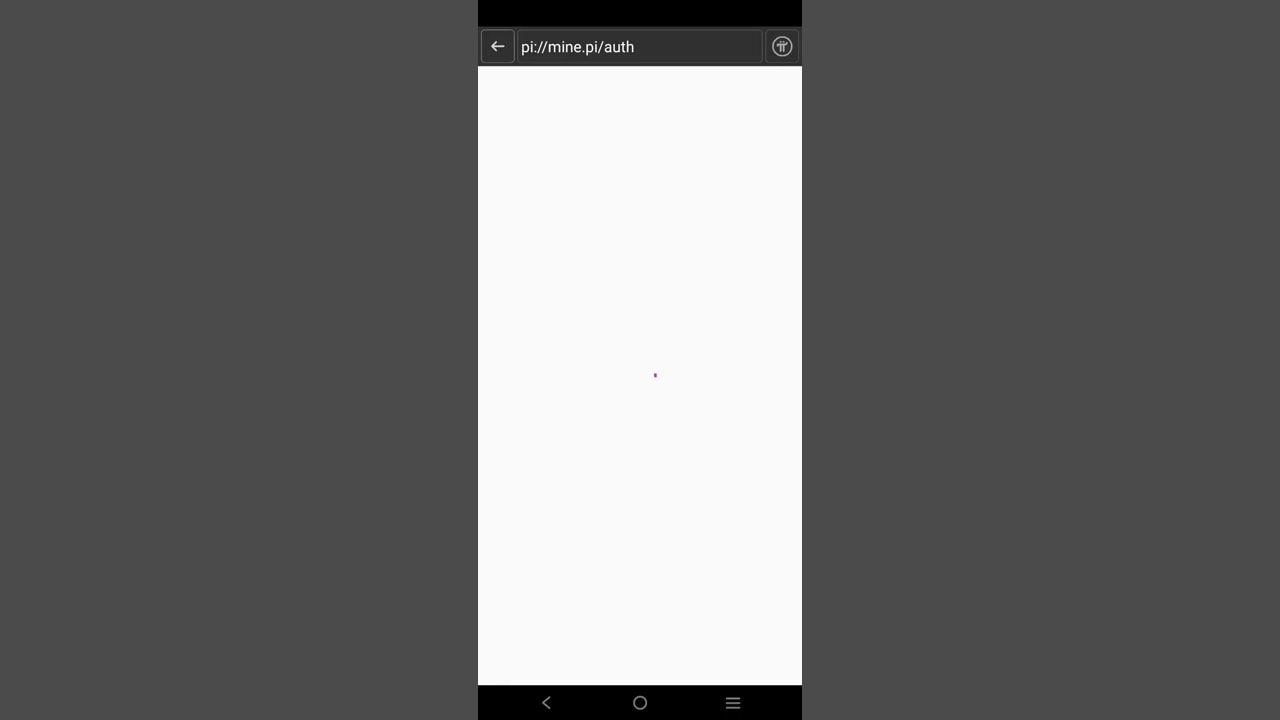The image features a screenshot of a phone displayed in the center of a horizontally rectangular frame with a white background. The phone's screen is entirely white, suggesting a possibly broken or blank web page. A horizontal black bar runs across both the top and bottom of the phone screen. Just below the top bar is a dark gray horizontal strip with a white left-pointing arrow and the text "PI;://MINE.PI/AUTH." The bottom black bar contains a similar left-pointing arrow on the left side, and a faint white circle in the center. On the right side of the bottom bar, there are three horizontally stacked white dash marks. The overall scene presents a minimalistic, somewhat non-functional digital interface against a plain background.